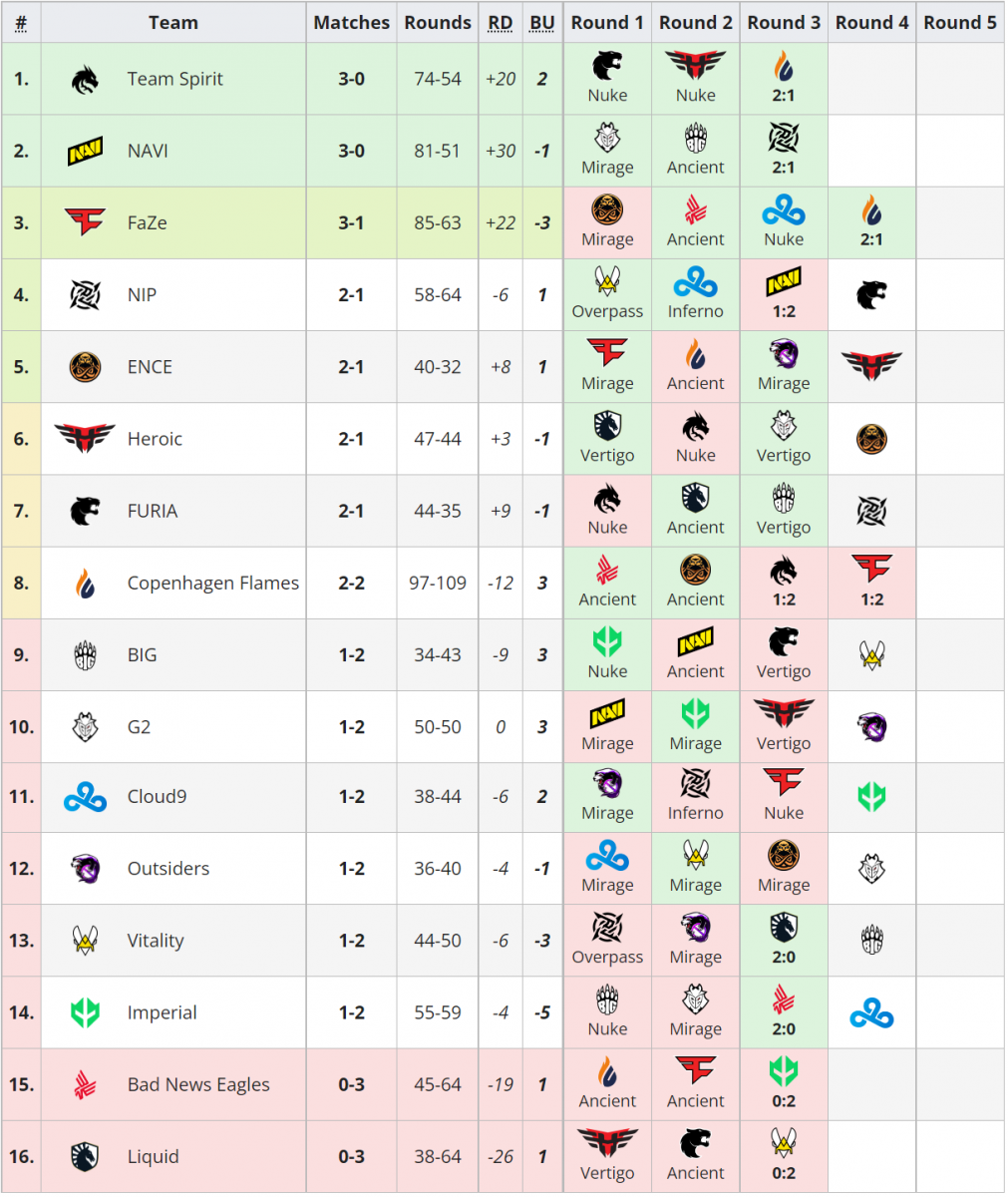This portrait-oriented image displays a detailed grid likely for a sporting event, listing teams, their opponents, and schedules. The header features a grey background with column titles. The columns, from left to right, are labeled as follows: Number (#), Team (centered in black font), Matches, Rounds, RD, BU, followed by Round 1 through Round 5. 

Teams are numbered 1 to 16, possibly indicating standings based on their records, with "Team Spirit" in the top position. Most teams have filled logos up to Round 3 and some up to Round 4, reflecting their schedules and opponents. 

The grid uses colors to differentiate outcomes: green signifies wins, pink indicates losses, and grey shades denote completed matches. Additionally, some teams are highlighted in light green and yellow, possibly to indicate special status or categories. 

"Team Spirit" and "Navi" are highlighted in green headers at the top, featuring unique icons or logos. A team named "Phase" is under a light green header, distinct from the others. Although the sport is not specified, this comprehensive grid provides a clear overview of team standings, schedules, and match outcomes.